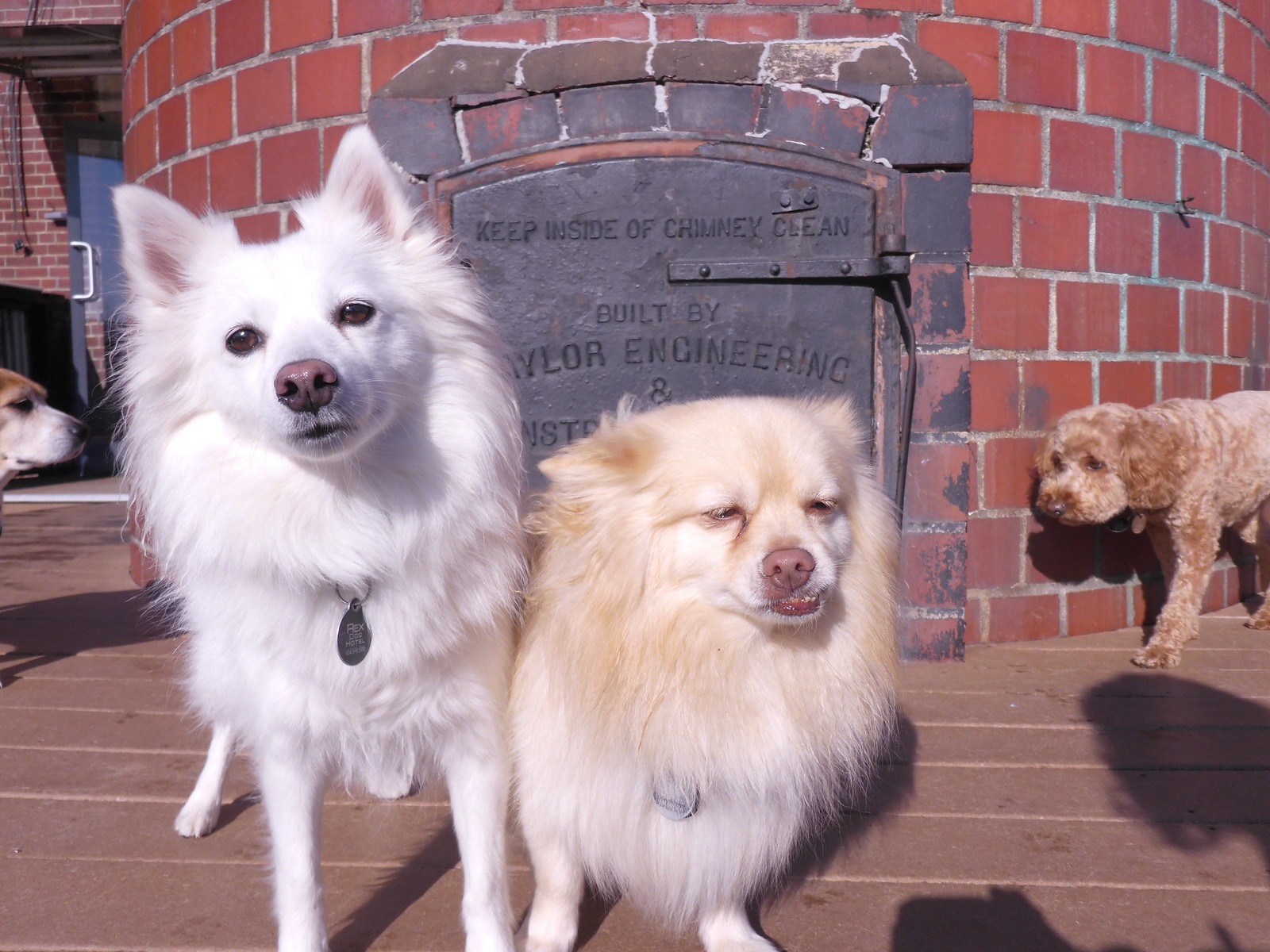The photograph captures four dogs standing around a rust-colored brick chimney with an engraved iron door that reads, "Keep inside of chimney clean, built by Taylor Engineering," though the dogs obscure additional details. 

In the center are two small, fluffy dogs resembling Pomeranians; the one on the left is entirely white with pointy ears and a red nose, wearing an oval gray dog tag. The dog to its right is a light tan with a mix of white, featuring downturned ears, and also wearing a partially obscured silver-gray tag. 

To the left is a partially visible face of a brown and white dog, likely a Beagle, while to the right stands a shaved-down Poodle with light brown curls around its ears and legs. They are all set against the backdrop of a wooden deck, casting shadows beneath them. In the background, the brick chimney forms a focal point, enclosed by additional brickwork, with a glass door and another brick wall visible to the left.